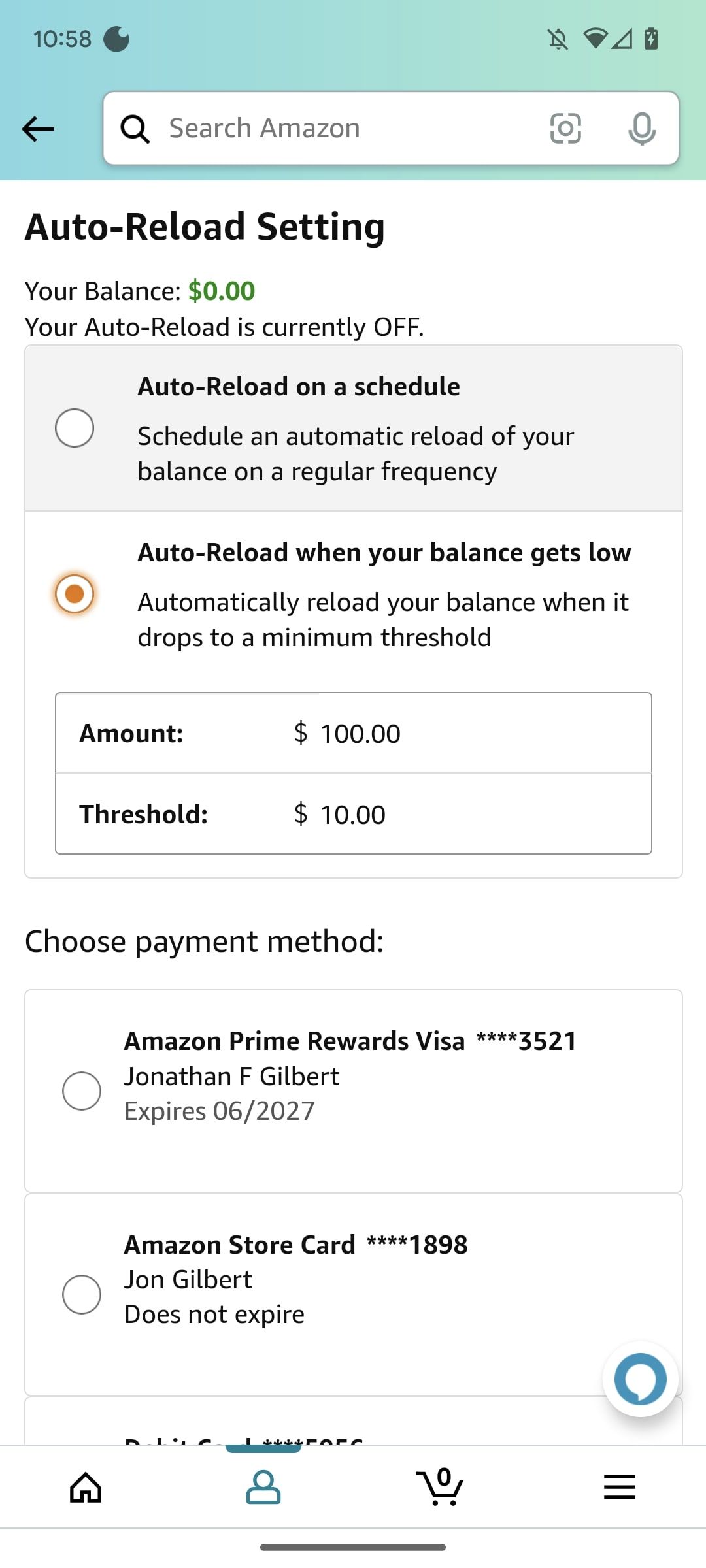The screenshot depicts an Amazon app interface. At the top, there's a blue banner displaying the Amazon logo on the left. Following the logo, it states "558." On the right-hand side, a crossed-out notification bell icon indicates no new notifications. Adjacent are icons for Wi-Fi, cellular data bars, and a battery icon showing charging status.

Below the blue banner, there's a search field with the placeholder text "Search Amazon." The main content sits on a white background.

Currently, it shows the auto-reload settings for an Amazon account. The text reads:
- "Your balance: $0.00"
- "Your auto-reload is currently off."

Two options are available for setting up auto-reload:
1. The first option, which is not selected, lets you schedule an automatic reload based on a regular frequency.
2. The second option, highlighted with an orange-checked circle, allows for automatic reloading when the balance drops to a specified minimum threshold. In this instance, the threshold is set at $10, and the reload amount is $100.

Underneath, payment methods are displayed:
- "Amazon Prime Rewards Visa," ending in 3521, belonging to Jonathan F. Gilbert, expiring in June 2027.
- "Amazon Store Card," ending in 1898, belonging to John Gilbert, with no expiration date.

Neither payment method is currently selected. 

In the bottom right corner, there's a teal-colored oval button with a white text bubble, while at the very bottom of the screen, navigation icons include a house, a person, a shopping cart with a "0" badge, and three horizontal lines representing a menu.